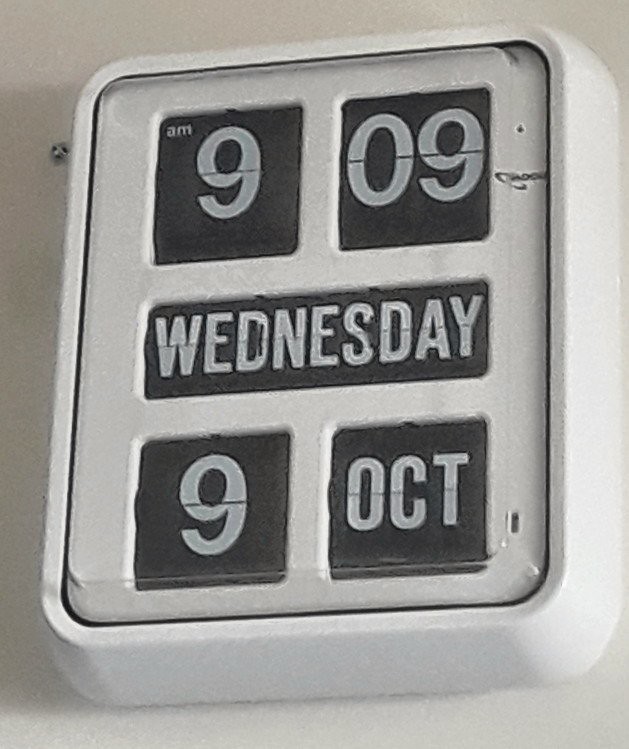Mounted on a white wall, the focal point is a digital clock with a unique mechanical flip design. The clock, which is rectangular in shape, indicates the time as 9:09. In the upper left-hand corner, there are designations for a.m. or p.m. Although the clock is digital, it does not utilize LED lights; instead, it employs a mechanical flipping mechanism. The brand name is present but indiscernible.

Below the time display, the day of the week is prominently featured in large white letters on a black background, which also flips to change. Further down, two separate boxes display the date and the month in abbreviated form, using black text on a white background, and these components are also designed to change mechanically.